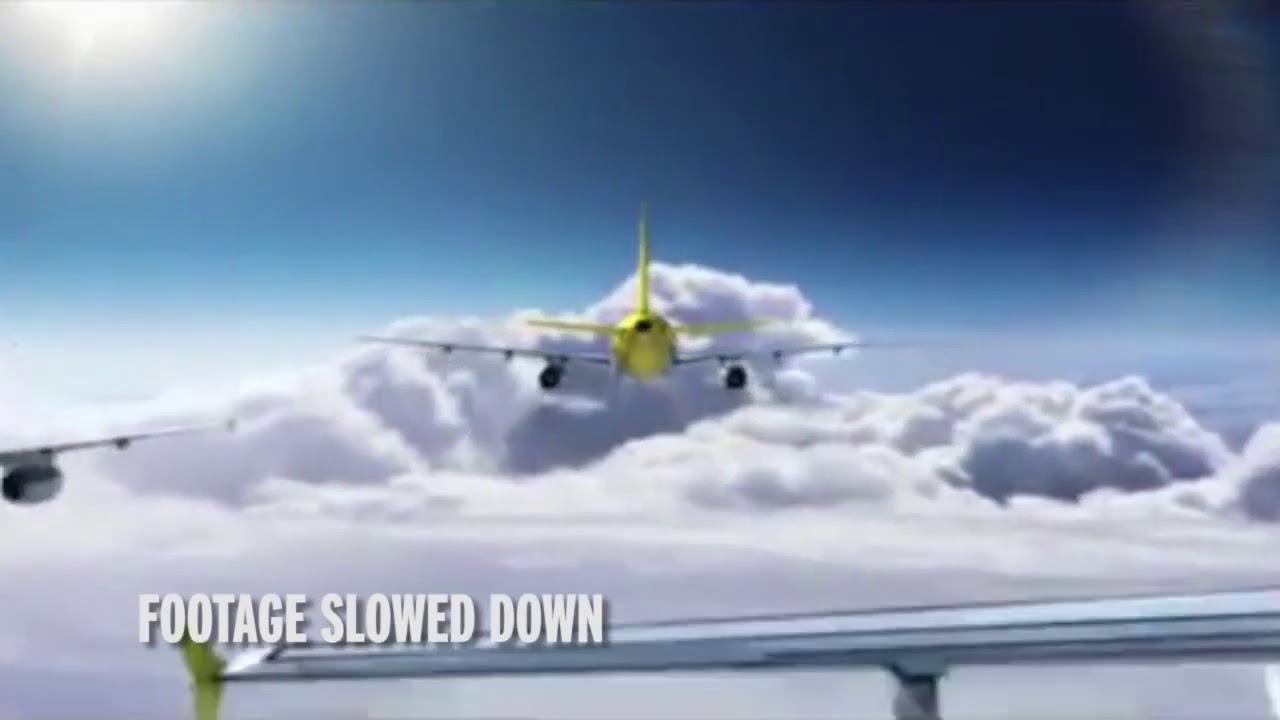The image captures a striking aerial scene featuring three large passenger airplanes flying in a triangular formation high above white, cumulus clouds against a vibrant blue sky with a prominent sun flare in the upper left corner. The centrally positioned plane is trailing lime green with gray wings, viewed from the rear, showcasing its tail wing and engines. Below, the full wing of another plane with a lime green tip and gray base spans across the bottom of the image. To the left, a partial gray wing of a third plane is visible. The entire scene highlights the close proximity of the aircraft, evoking an impressive but precarious formation flying scenario. Overlaid at the bottom left of the image, in all capital letters, "FOOTAGE SLOWED DOWN" is printed in white text with a drop shadow, suggesting the dynamic nature of the captured moment. The clear sky and clouds beneath the planes enhance the dramatic and serene aspects of the photograph.